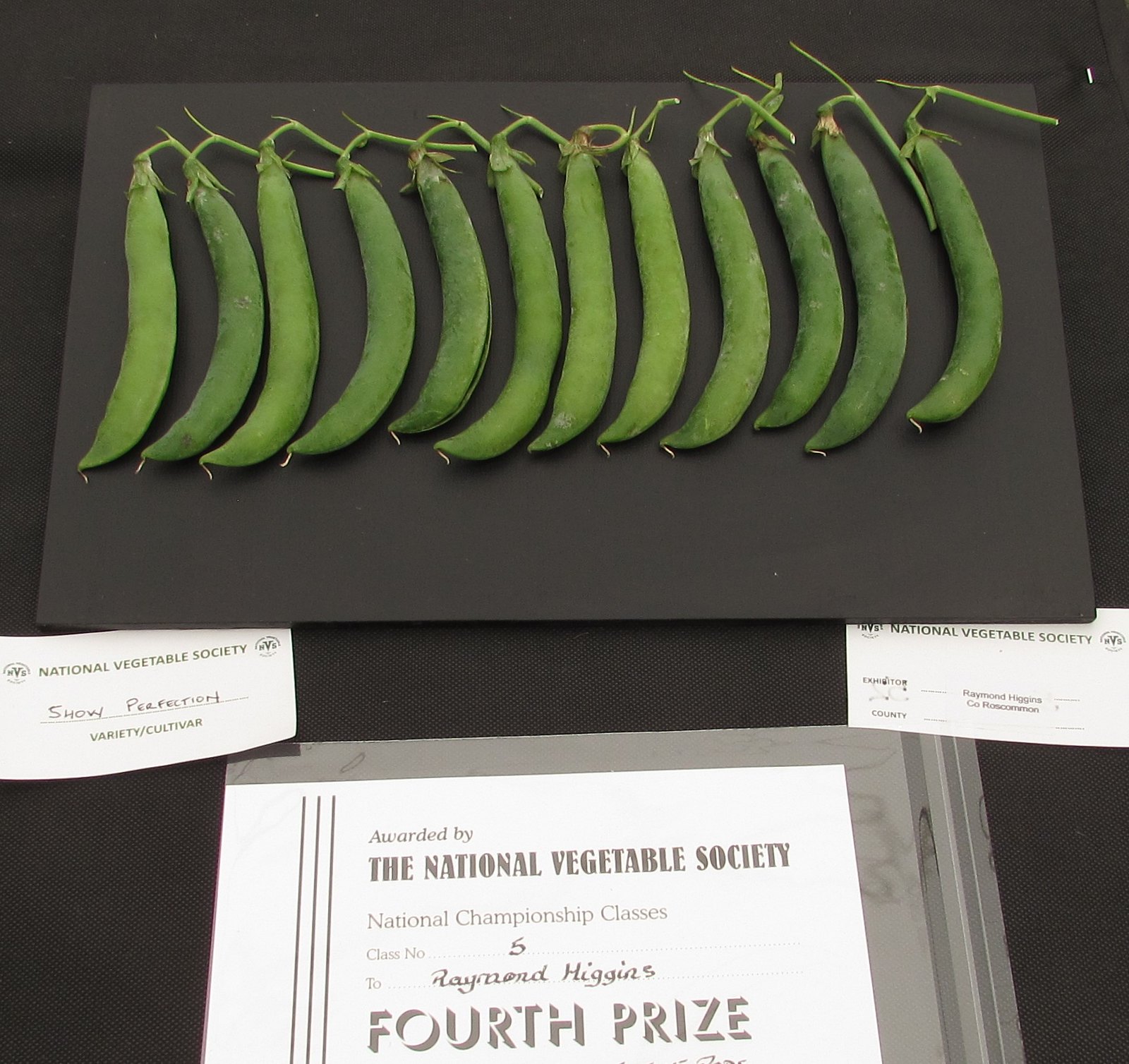This image showcases a display from a National Vegetable Society contest. The focal point is a row of 12 freshly picked green beans, displayed horizontally on a black rectangular platform, with each curved to the left. Beneath the beans lies a white and silver certificate that reads, "Awarded by the National Vegetable Society, National Championship Classes, Class Number 5, to Raymond Higgins, Fourth Prize." Additionally, there are two smaller pieces of paper positioned to the lower left and right of the platform, both adorned with the National Vegetable Society's name and some hand-written details, though these are illegible from the photograph. The overall background is black, making the green beans and certificates stand out prominently.